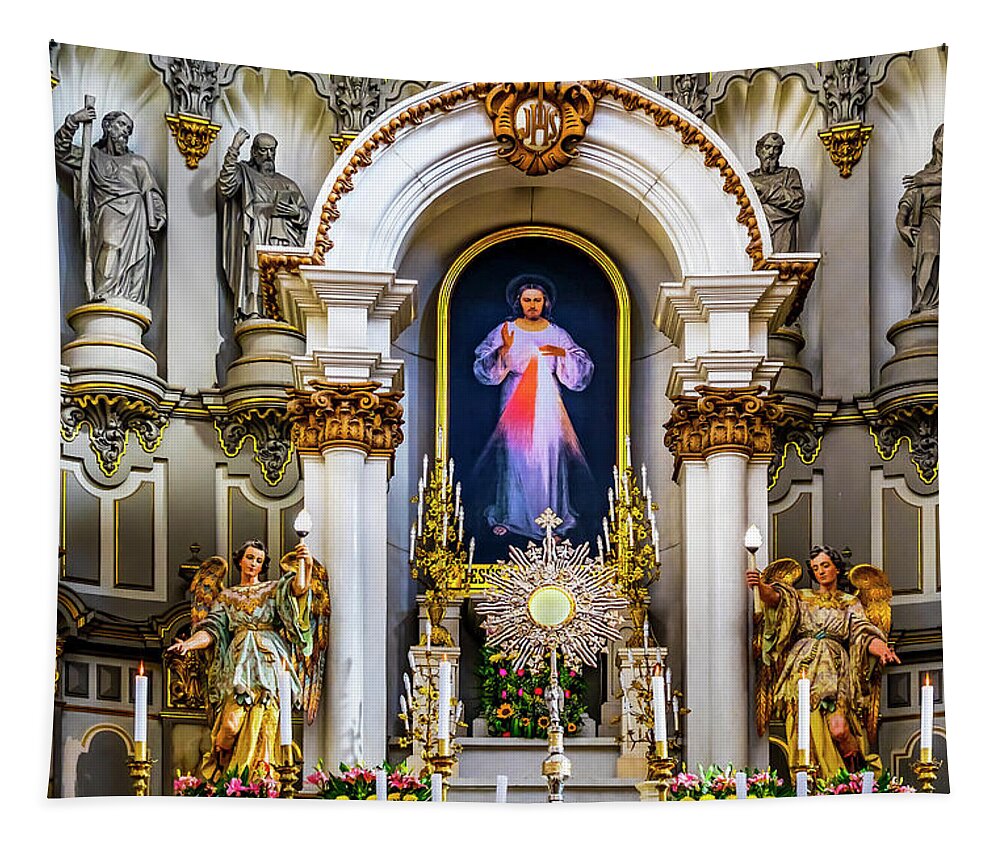The image depicts a sumptuous church interior with a central altar surrounded by ornate arches. At the heart of the altar is a prominently displayed picture of Jesus, beneath which the word "Jesus" is inscribed in a large golden frame. The scene is bathed in a bright, almost ethereal light that enhances the antique setting, dominated by white, brown, gold hues, and intricate marble work. Numerous white candles and pink flowers adorn the space, contributing to its majestic ambiance. Two angels, positioned symmetrically on either side of the altar and holding lights, stand guard before rows of additional candles and flowers. Flanking the altar are statues of four men, possibly apostles, each depicted in a different pose: one holding a stick and gazing at Jesus, another reading from a book with his fist raised, a third folding his arms, and the last only partially visible. The overall scene is rich with historical and religious symbolism, creating a sense of awe and reverence, yet there is an overdone, almost too-perfect quality that raises questions about whether the image is an actual photograph or an AI-generated visualization of a church.